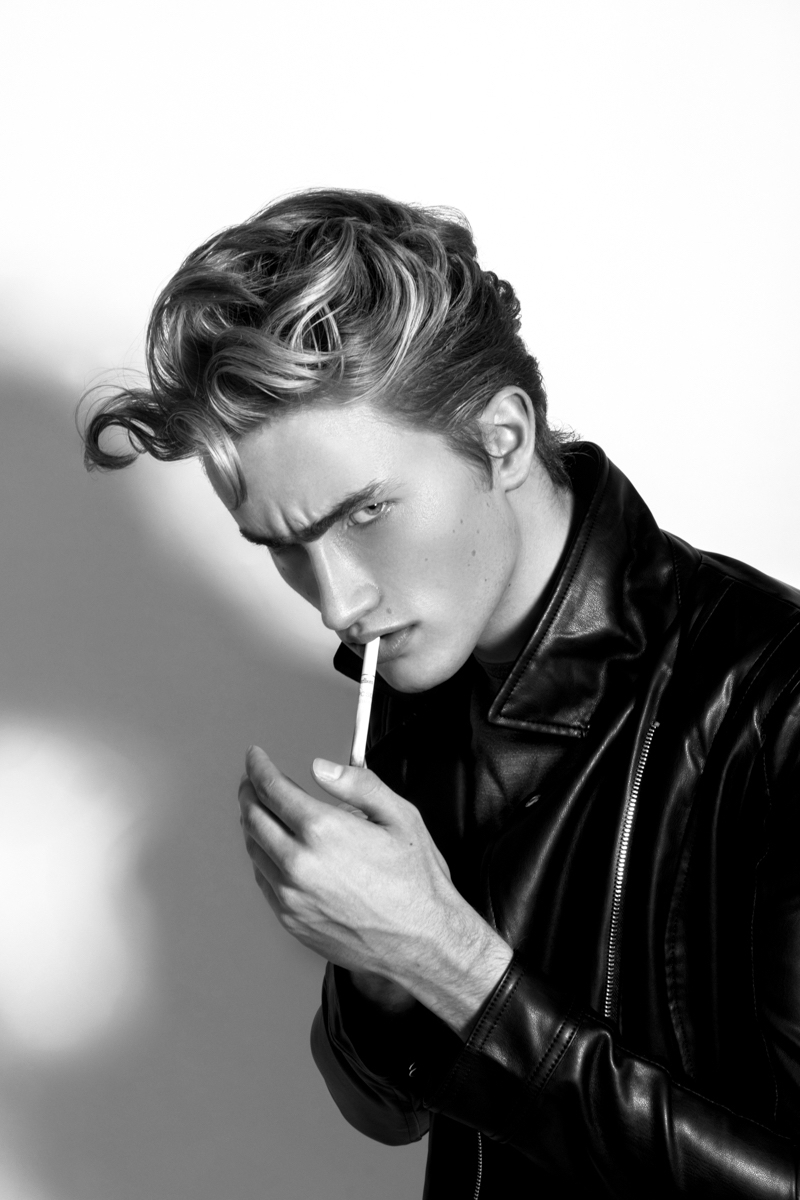In this evocative black and white photograph, model Dylan Berloui masterfully channels the iconic look of James Dean. The image captures the upper half of his body, clad in a black leather jacket with distinctive zippers and a turned-up collar. Berloui's hair, blonde and styled in curled swirls on top, adds to the nostalgic flair of the piece. With his head slightly tilted down and his furrowed brow, he stares intensely into the camera, eyes angled upward in a serious, almost brooding expression. He holds a cigarette in his mouth, one hand poised to light it with a lighter while the other steadies the cigarette. The background is a light gray or off-white, highlighted by the subtle shadow he casts against it. Berloui’s pose and attire meticulously evoke the rebellious spirit of James Dean, making this photograph a compelling homage to the legendary actor.